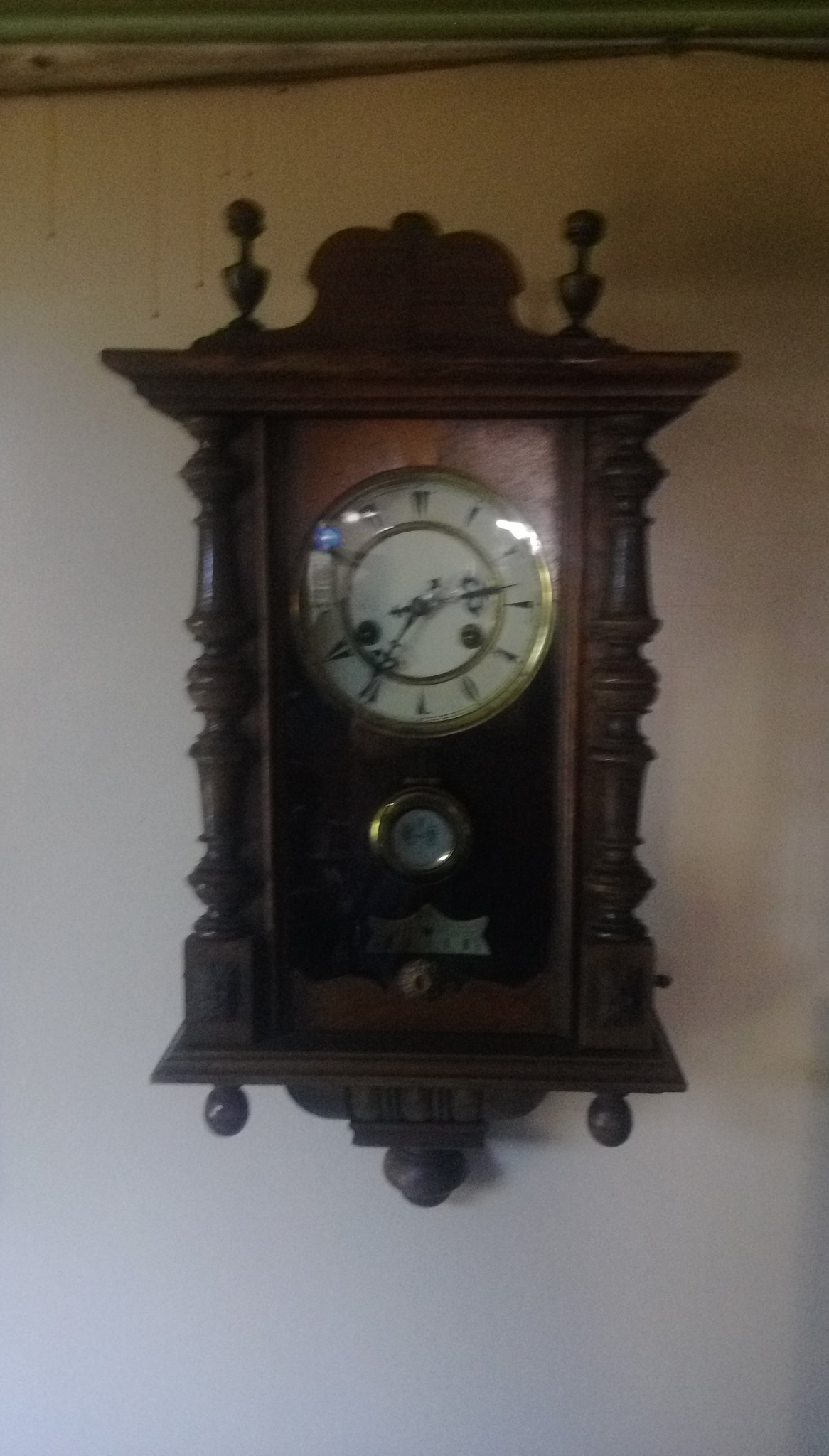An ornate clock hangs prominently on a white wall. The case of the clock is crafted from dark wood, shaped into an upright rectangular form. It features elaborate details, including a platform top and a decorative bottom, both adorned with lathe-turned pillars on either side and extending above and below the main body for added embellishment. The clock face is a creamy white, encircled by two concentric gold rings—an outer and an inner one. Instead of traditional numbers, it has simple dashes marking each hour and every five-minute increment. Two intricate black hands point to the current time of 2:35. Below the clock face, there's a round, gold-colored circle with a gray interior, the purpose of which remains unclear. This elegant timepiece, with its detailed craftsmanship, stands out beautifully against its stark background.